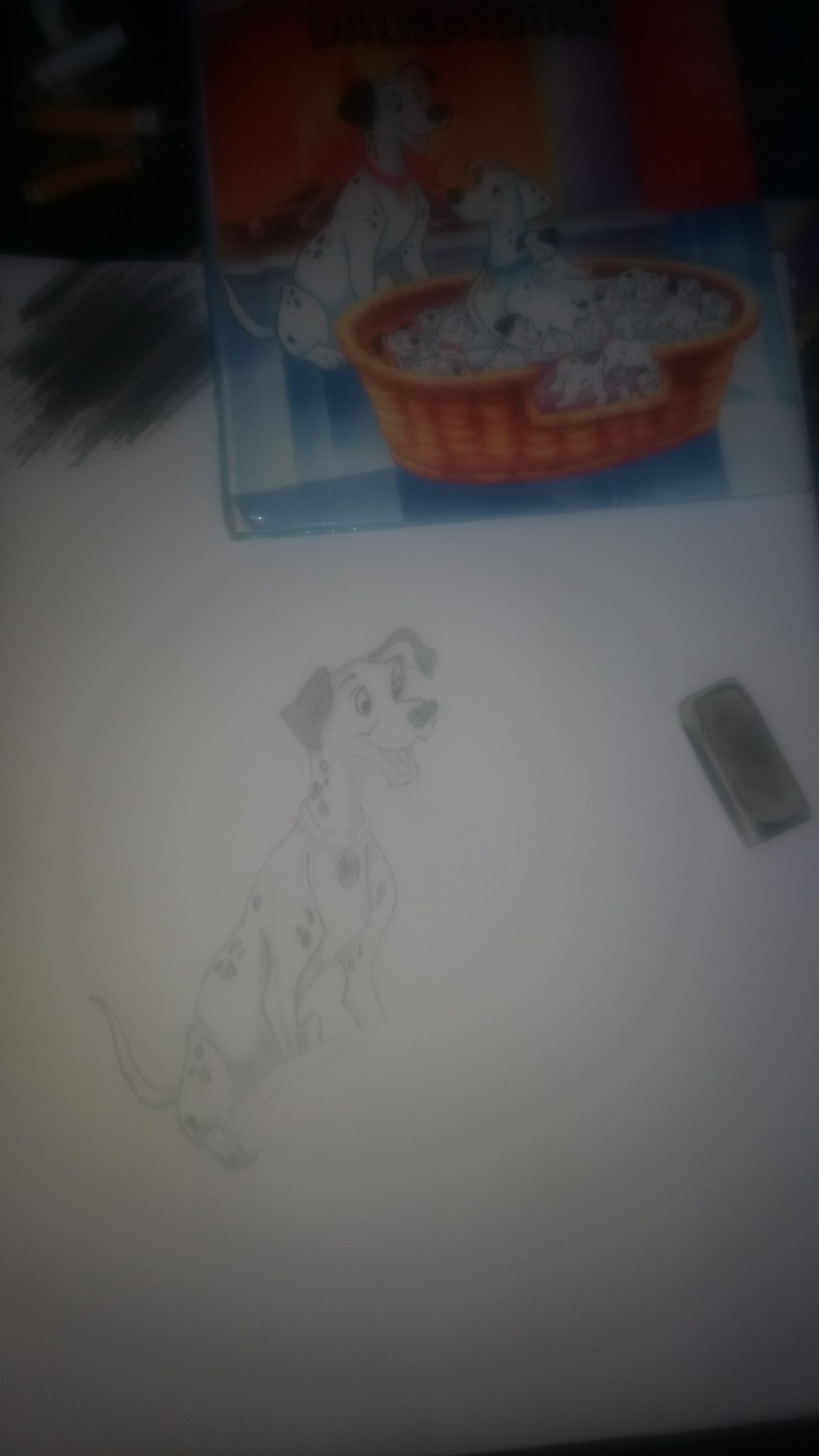In this blurred color photograph of a sketch, the artist has drawn a detailed pencil image of a Dalmatian from Disney's 101 Dalmatians on a white piece of paper. The long rectangular sketch is positioned centrally towards the left side, with the Dalmatian's face turned to the right, showcasing its black nose, floppy ears, and a smile with its mouth open. Black spots cover the dog's white fur, and it wears a circular symbol around its neck. To the right of the sketch, near the center, is a gray eraser lying on the paper.

At the top center of the photo, an official color image from the 101 Dalmatians movie is pinned, depicting the male Dalmatian looking at a large brown basket filled with the mother dog surrounded by numerous puppies. The top left corner of the photo reveals thick pencil scribbles where the artist experimented with shading, and next to it, some chalk sticks rest on a dark surface. The right side of the photo, particularly the bottom right, fades into darkness, highlighting the contrast between the paper and its surroundings.